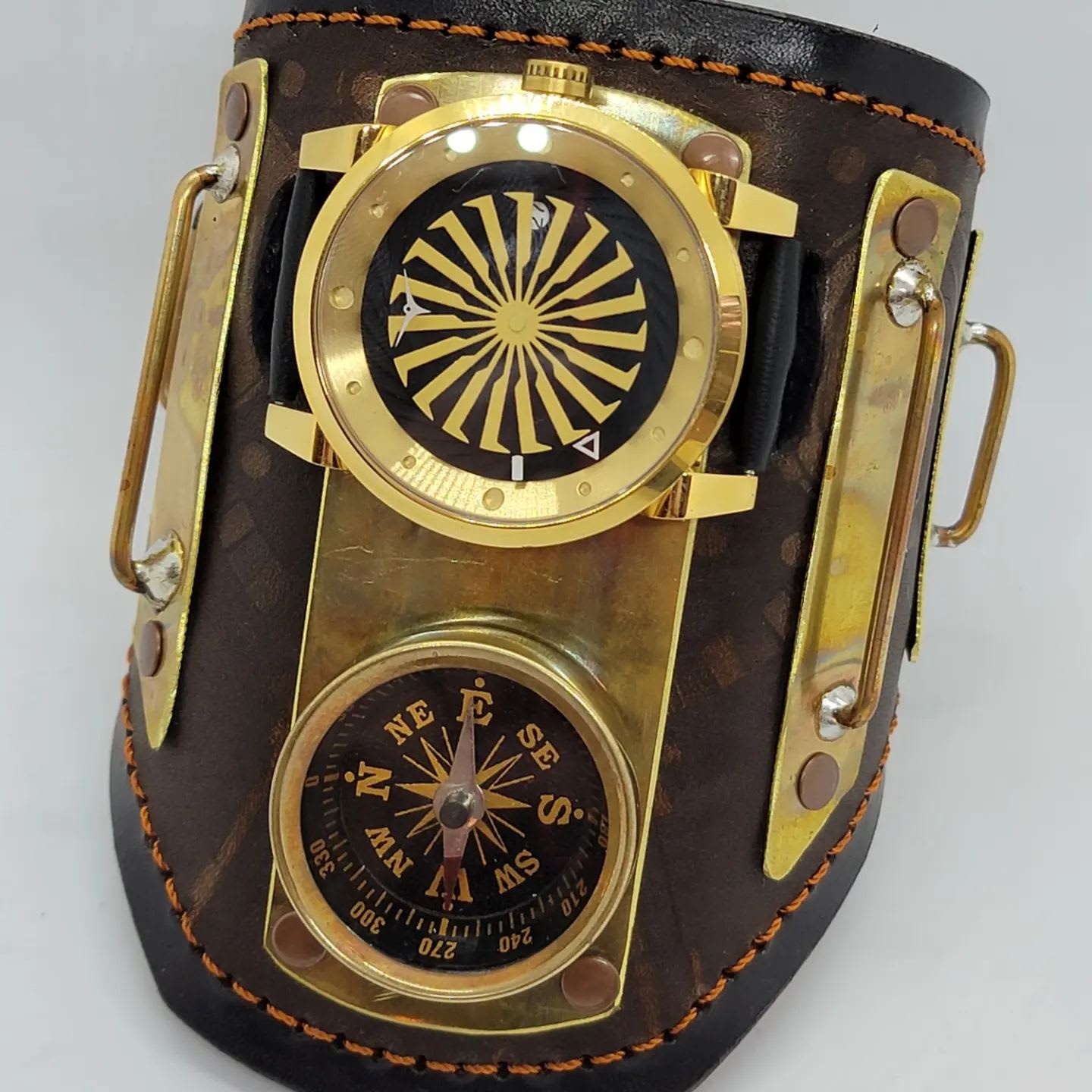The image displays a detailed, brown leather wrist guard set against an all-white, slightly gray background. The wrist guard features intricate brown stitching and is adorned with various gold metal elements. Prominently, it has two circular compasses mounted on it: one at the bottom and one at the top. The bottom compass has a black background with gold lettering indicating the cardinal directions (North, South, East, West) and intermediate points (Northeast, Northwest, Southeast, Southwest), as well as numbers ranging from 0 to 330. The compass hand itself is silver. Above this, there is another circular feature resembling a compass, but instead of letters and numbers, it contains an image of the Sun and lacks a directional hand. Both of these elements are mounted on gold platforms, enhancing the aesthetic appeal of the wrist guard. This descriptive and clear image is brightly lit, showcasing its vivid colors and intricate details.